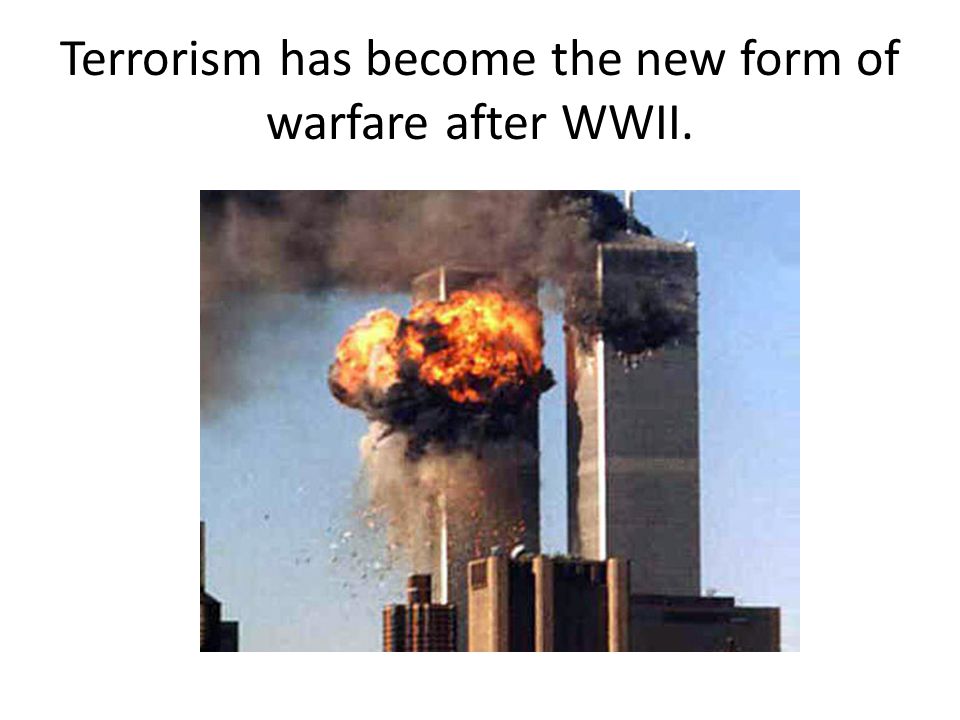The image features a powerful color photograph set against a white background, directed to convey a profound message about modern terrorism. At the top of the image, in a centered sans serif font, the headline reads, "Terrorism has become the new form of warfare after WWII," emphasizing a shift in global conflict post-World War II. Below the text, the photo captures a moment from the September 11th, 2001 attacks on the Twin Towers in New York City. The twin towers, severely damaged, dominate the scene. On the left, a massive burst of fire and an explosion can be seen, with smoke and debris foregrounded against a clear, powder blue sky to the right, creating a stark contrast between the chaos and the calmness of the day. The image is photorepresentational and might be used in an online article, a presentation, a newspaper, or an awareness campaign, evoking the abrupt transition from peace to destruction in moments of terror. The colors black, gray, blue, red, orange, and yellow highlight the intense and tragic nature of the scene.